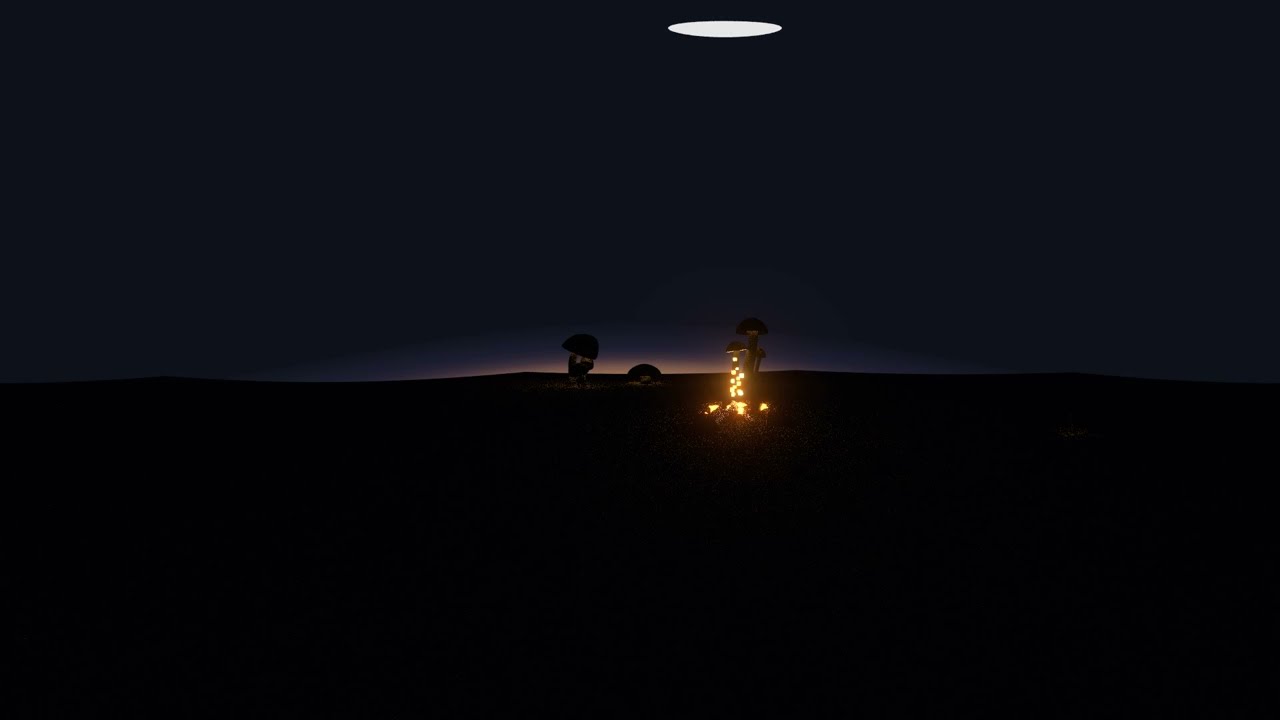This is a rectangular horizontal nighttime photograph characterized by its dark and mysterious ambiance. The sky above is a deep purple, almost bluish in some perspectives, lending a surreal quality to the scene. The most striking feature is in the center-right of the image, where three tall, mushroom-shaped objects stand prominently. These objects are illuminated, with light emanating from the caps down to their bases, creating a stark contrast against the surrounding darkness. The leftmost mushroom appears especially bright.

The terrain below these objects is shrouded in darkness, suggesting a vast, flat expanse that could resemble a desert or a mountainous area. This combination of illuminated mushrooms and the dark, expansive foreground gives an impression of a futuristic or otherworldly landscape. The photograph also features a disc-like object at the top, initially mistakable for the moon but also evoking the image of a flying saucer, adding to the enigmatic atmosphere of the scene.

In summary, the image captures a surreal nighttime landscape with illuminated, mushroom-like structures rising from a dark, expansive ground underneath a purple sky, all augmented by an eerie, disc-shaped object above.